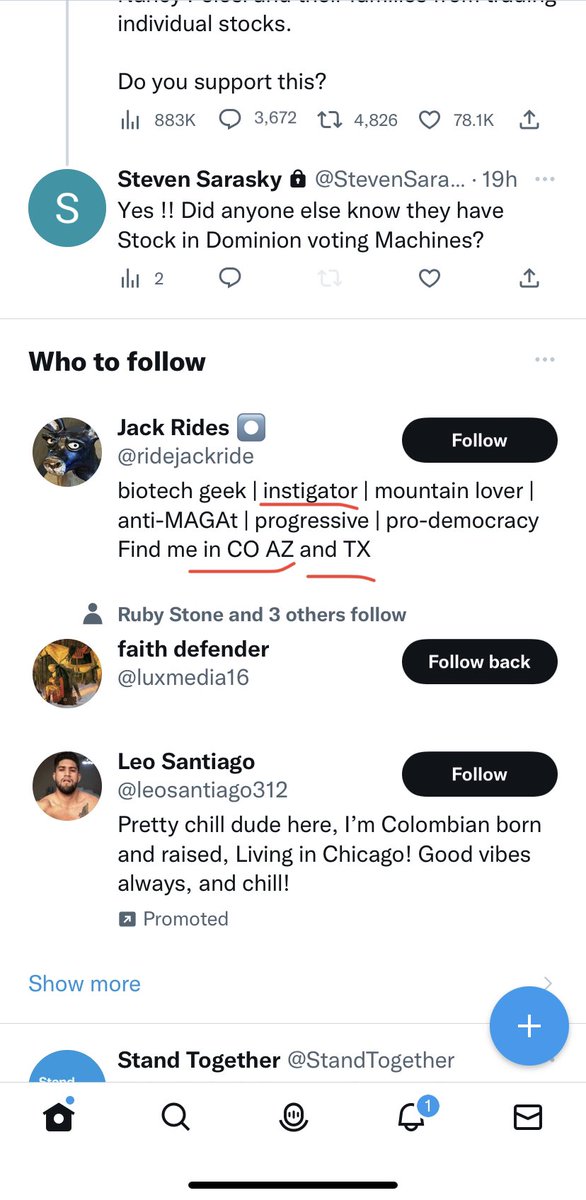The image appears to be a cropped screenshot of a tweet. The top part of the image is partially cut off, showing only the words "individual stocks." Below this, there is a question asking, "Do you support this?", followed by a response from Steven Sarosky stating, "Yes, did anyone else know they have stock in Dominion Voting Machines?". 

Steven Sarosky’s profile image features a green circle with an 'S' inside. Below his tweet, there's a "Who to follow" section listing Jack Rods, who has a dog in his profile picture. Jack Rods’ handle is '@rideJackRod' and his descriptive bio reads: "biotech geek," with "instigator" underlined in red, followed by "mountain lover," "anti-MAGA-T," "progressive pro-democracy," and "find me in NOCOAZNTX," with the E in "find me" and "NOCOAZNTX" also underlined in red.

The overall style of the image suggests it's from a social media platform.